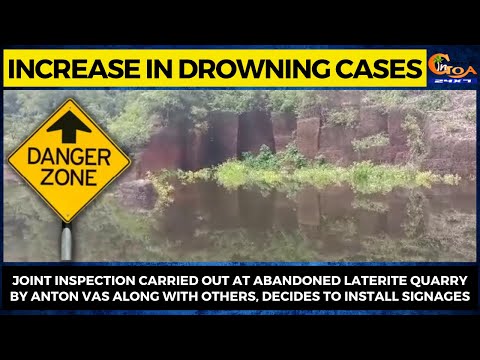A news feed photograph, bordered in dark black with a bright yellow section at the top reading "Increase in Drowning Cases," depicts a dangerous area at an abandoned laterite quarry. A prominent diamond-shaped yellow sign in the middle of the image displays "Danger Zone" with a black arrow pointing up. The quarry features clay-colored stone structures interspersed with grass and moss, suggesting the presence of hazardous terrain and water. The caption under the photo reads, "Joint inspection carried out at abandoned laterite quarry by Anton Voss, along with others, decides to install signages," highlighting the efforts to improve safety by placing warning signs in response to the rising number of drowning incidents in Goa.